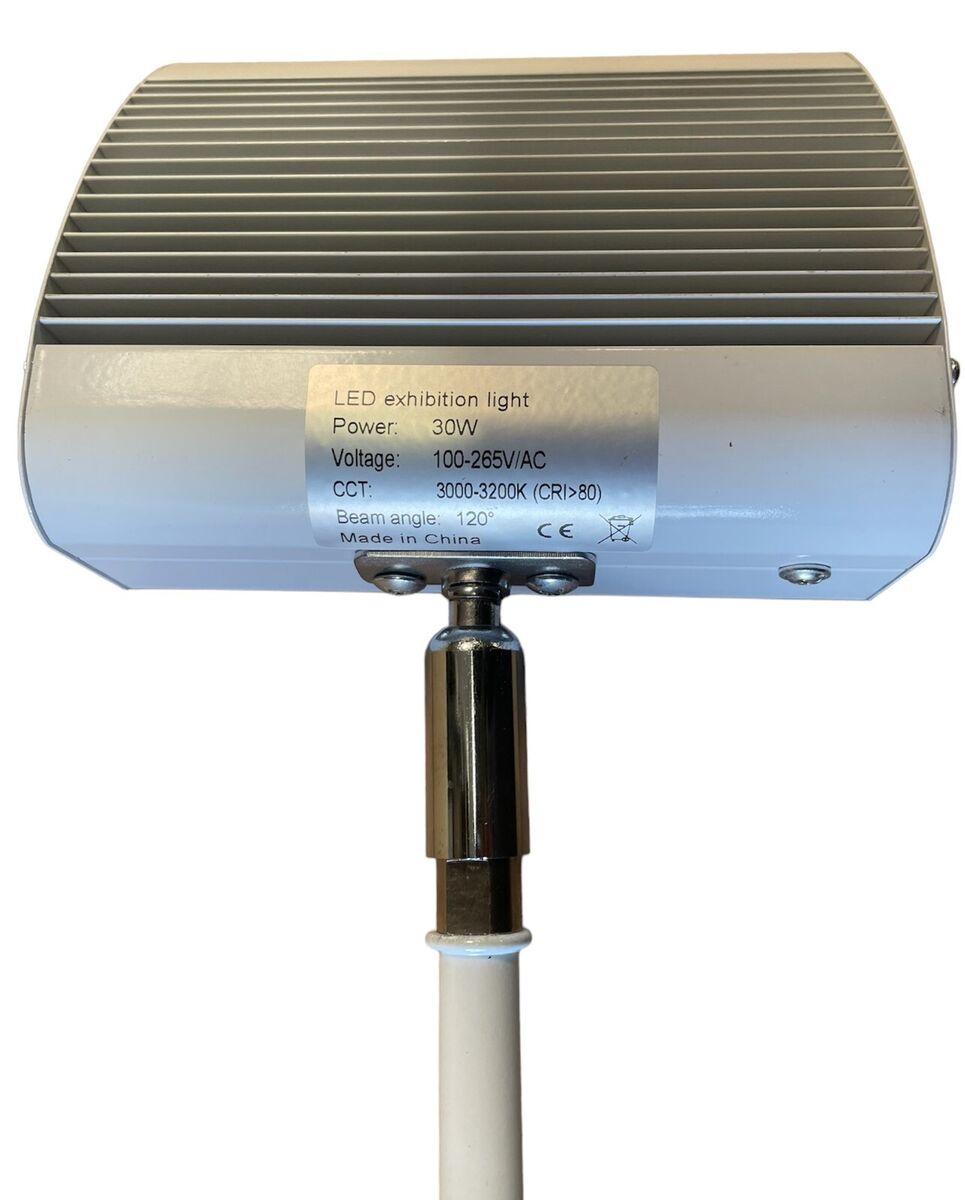The image depicts an LED exhibition light positioned against a stark white background. This rather old-looking light features a prominent metal pole that extends down into the base, secured by two screws on either side. The design includes the large LED light fixture on top, resembling an air conditioning unit with visible rays, suggesting where the lights emit from. 

Notably, there’s a detailed label affixed to the light, specifying key technical details: “LED Exhibition Light” with a power rating of 30 watts, a voltage range of 100 to 265 volts AC, and a CCT (Correlated Color Temperature) between 3,000 to 3,200 K. The label also mentions a CRI (Color Rendering Index) greater than 80, a 120-degree beam angle, and notes that it was made in China. The label includes an icon indicating that the product is non-recyclable. The pole supporting the light is half white and half metal, complementing the overall industrial aesthetic of the exhibition light.